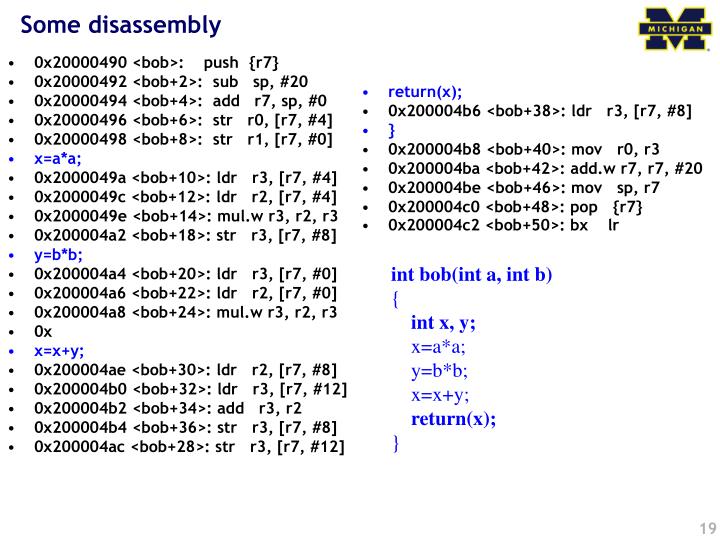The image depicts a detailed slide focused on disassembly code, set against a white background. The top right corner features the University of Michigan logo, characterized by a large blue "M" with the word "Michigan" across it, accented by yellow and gold outlines. In the upper left corner, the text "SOME Disassembly" is prominently displayed in blue. The slide is densely populated with multiple lines of code and mathematical formulas, each line typically starting with "0x" followed by various numbers and commands. Interspersed among the black bullet points are blue lines highlighting key mathematical operations such as "x = a * a" and "y = b * b." The page is organized with code lines aligned on both the left and right sides, featuring a mix of black and blue text. Notable commands include "initbob," "inita," "initb," and "return." The bottom right corner marks it as page number 19, suggesting it is part of a larger manual or textbook, likely used in a higher education setting.